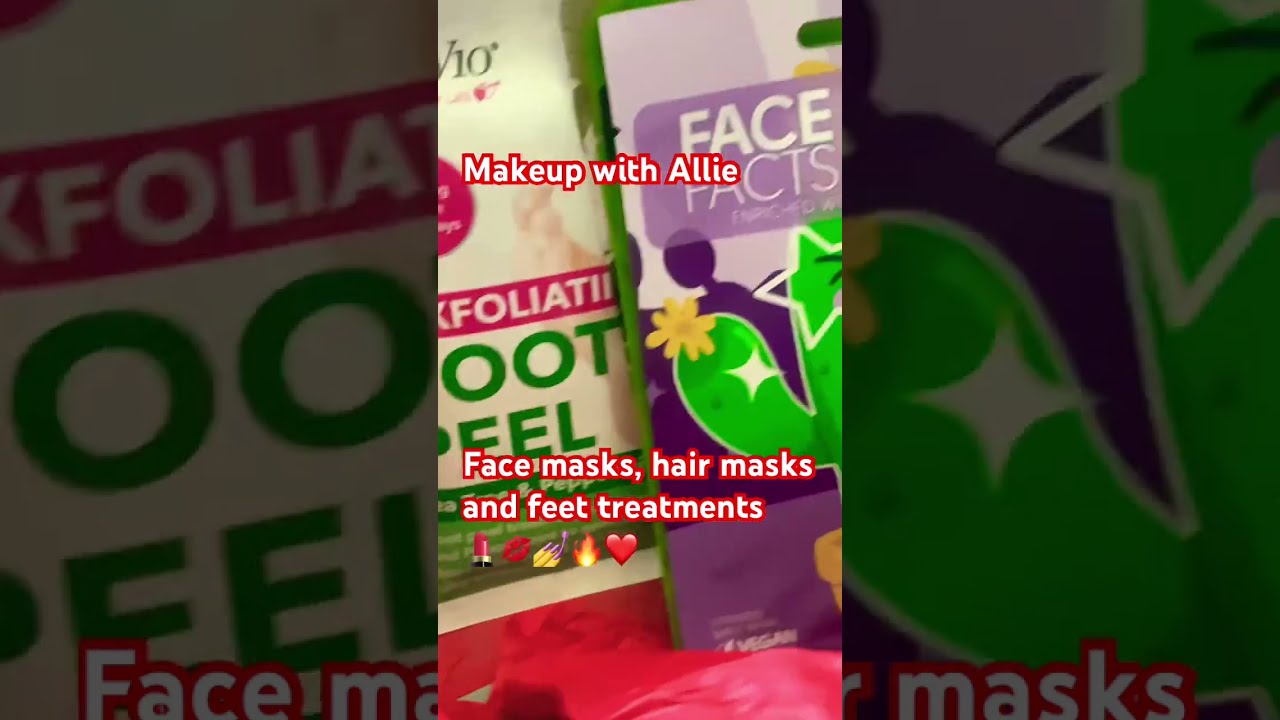This image is a detailed and elaborately edited landscape-style photograph, potentially a still from a video, showcasing two personal care product packages in the center, flanked by mirrored, grayed-out segments of the same image. The primary product on the left features a white base with pink accents and prominent green text that suggests it might be an exfoliating foot peel. The right product is encased in purple packaging adorned with a green cartoon cactus and the partially visible brand name "Face Facts." Both packages rest on a pink surface. Overlaying the entire image is text in a white sans-serif font with a red border, reading "Makeup with Allie," and underneath that, "Face Masks, Hair Masks, and Feet Treatments," accompanied by a series of emojis: Lipstick, Lips, Paint Nails, Fire, and Heart.